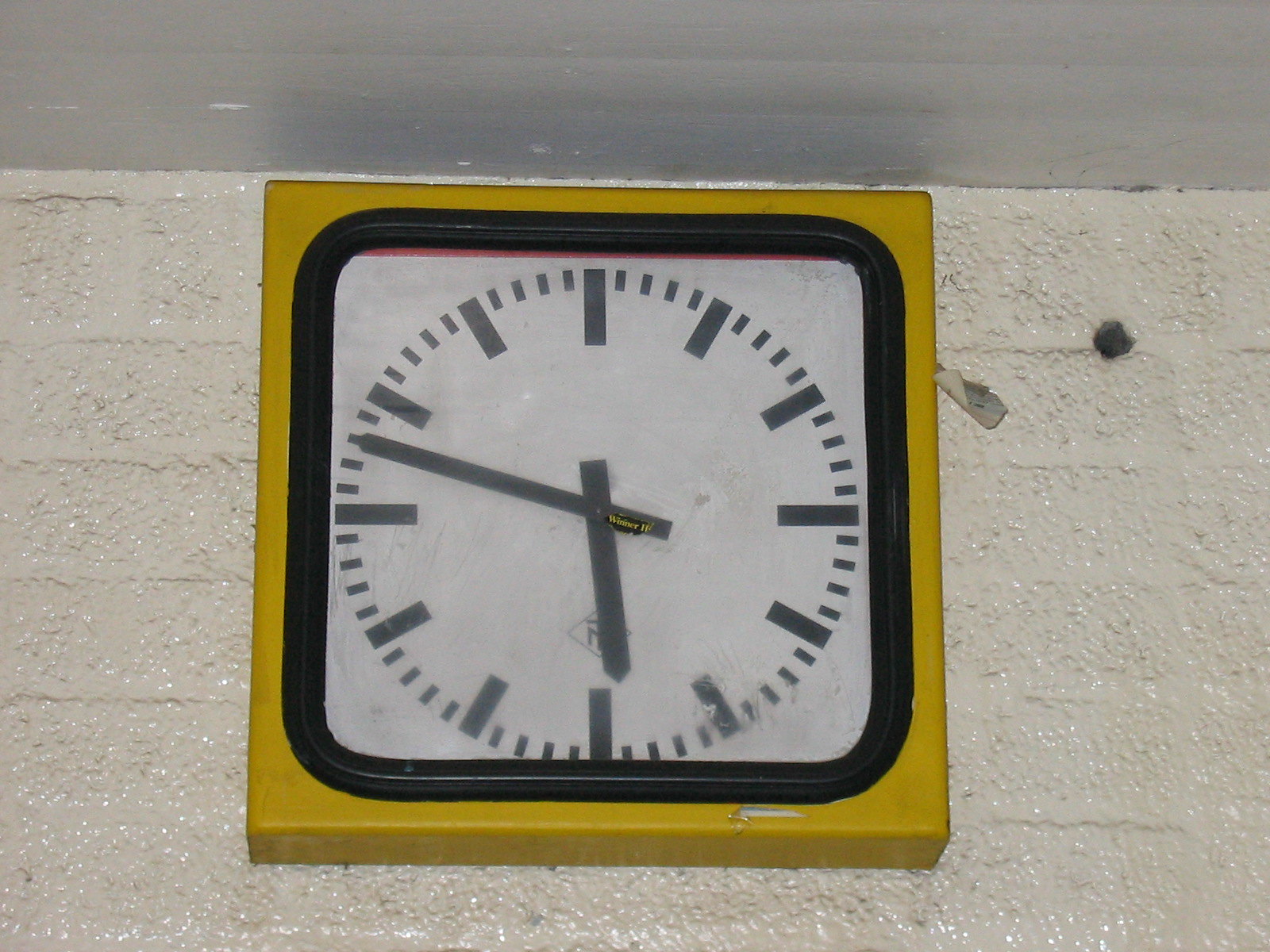A close-up image captures a square clock mounted high on a stark, white concrete wall, positioned just below the white ceiling. The clock features a two-toned frame: an outer yellow border and an inner black, rubbery plastic frame, both maintaining the square shape. Inside the clock, the design transitions to a circular format, marked with minimalistic black notches for hours and minutes on a white background. The hour marks are distinguished by long rectangles, twice the thickness of the smaller, slender minute marks. Notably devoid of numbers, the clock displays the precise time of 5:48 with its black hour and minute hands. The corners of the square clock face remain plain, creating a sharp contrast against the detailed circular display within.